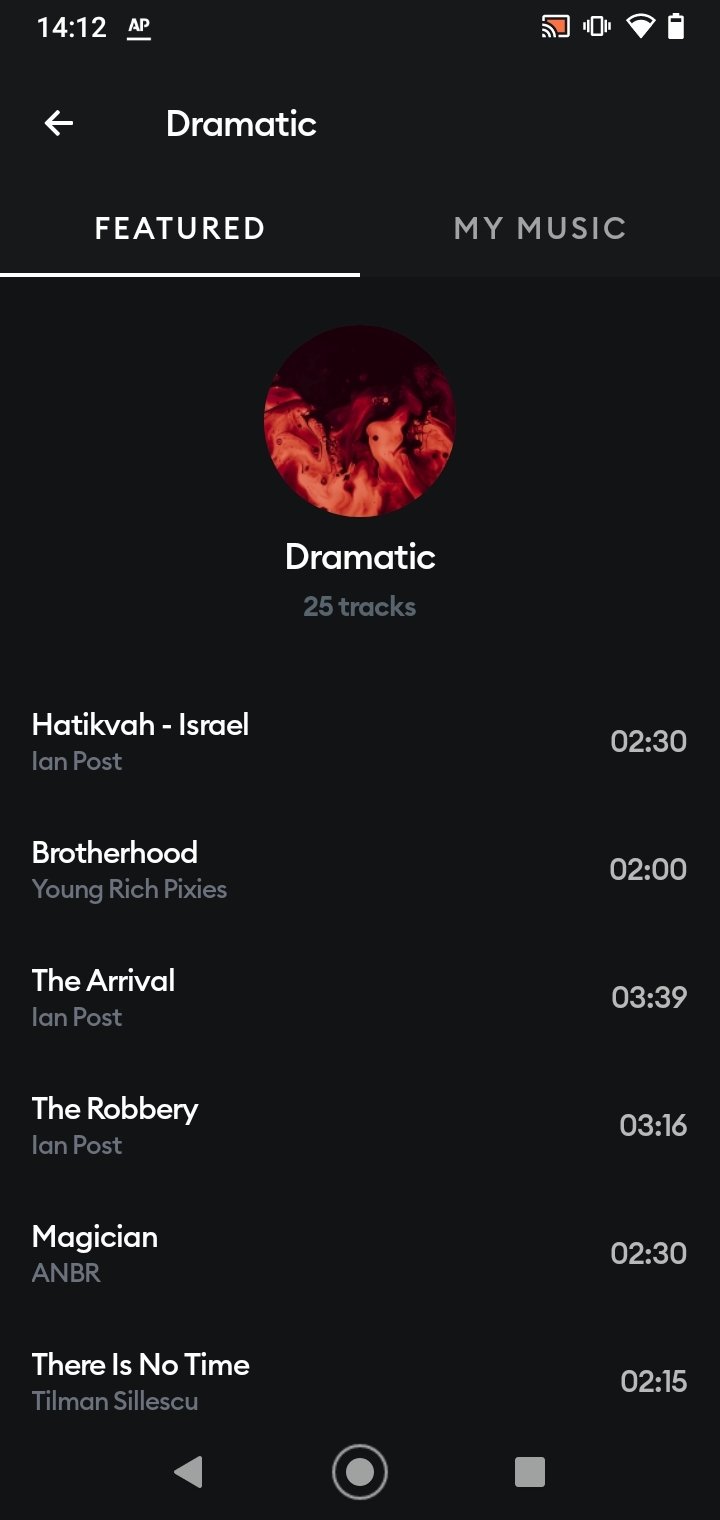The image displays a vertically oriented rectangular box with a black background and white text throughout. In the top left corner, the time is shown as "14:12." To the right of the time, the letters "AP" are underlined. Moving further to the right, a multicast symbol is present.

The phone is on vibrate mode, indicated by the corresponding icon, and the Wi-Fi signal shows three or four bars of strength. The battery icon suggests that the battery is nearly full, but not completely charged.

Below this top row, on the left side, an arrow points to the right next to the word "Dramatic" in white text. Below "Dramatic," the text "Featured in My Music" appears, with "Featured" underlined and slightly brighter than "My Music."

Continuing down the image, there is a circular icon with red flame-like visuals. Centered beneath this icon, the word "Dramatic" is displayed again, along with "25 tracks" in smaller text.

Further down and aligned to the left, the text "Hadikva-Israel" appears, with "Ian Post" written underneath it. This is followed by the duration "2 minutes and 30 seconds." Still on the left side, another entry reads "Brotherhood-Young Rich Pixies," with a duration of "2 minutes" displayed on the right.

At the bottom, the text "The Arrival by Ian Post" is noted, with the duration "3 minutes and 39 seconds" on the right side.